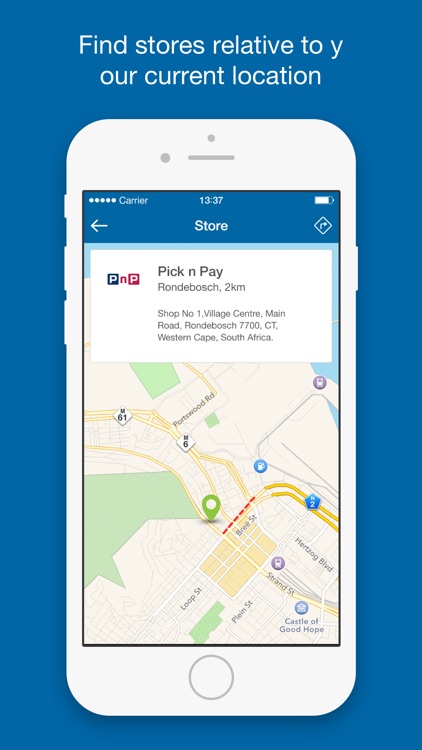The image features a vertical blue rectangle with superimposed white text that reads, "Find stores relative to our current location." The text capitalizes the first letter, ‘F’. Beneath this blue rectangle, there appears the outline of a white smartphone. Within the smartphone's screen, a detailed map is displayed. At the very top of the smartphone screen, a blue bar indicates the carrier, time, and battery life—specifically showing the time as 13:37.

Below the blue bar, the heading "Store," accompanied by a back button is prominently displayed. Positioned on the map at the top portion of the screen, there is a white rectangle. Inside this white rectangle on the top left side is a logo labeled "PNP." The logo is broken down into blue for 'P', red for 'N', and red for the subsequent 'P', which represents "Pick and Pay." Below the logo, it mentions "Pick and Pay Rondebosch," indicating it is 2km away, located in shop number 1 at Village Centre on Main Road, Rondebosch 7700 CT, Western Cape, South Africa. The map continues to be visible beneath this white rectangle.